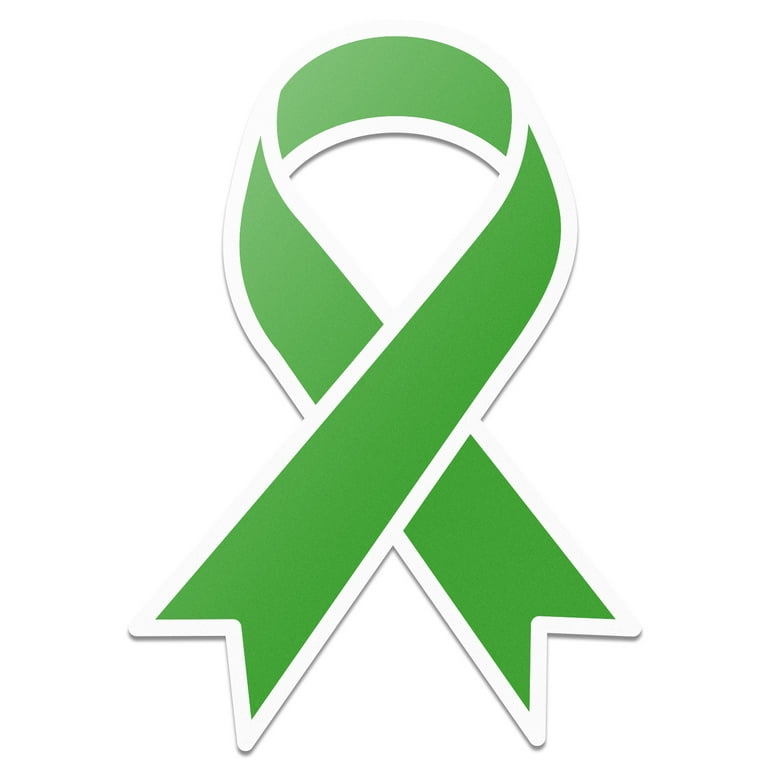The image showcases a green awareness ribbon with a crisp white outline, sitting prominently against a plain white background. The ribbon forms a classic loop, starting from the left bottom corner, routing upwards to the right top corner, before bending over itself and descending back to meet the bottom right. The ribbon's ends are notched with inverted triangles, giving them a spiked appearance. Encircling the green center is a thin black border, adding a subtle frame to the piece. The ribbon is perfectly centered in the image, with both ends meeting symmetrically at the bottom. The white border between the black outline and the green ribbon enhances its distinct shape, emphasizing its flat, sticker-like appearance. This green ribbon is commonly associated with various awareness campaigns akin to the pink ribbons for breast cancer or yellow ribbons to support the troops.